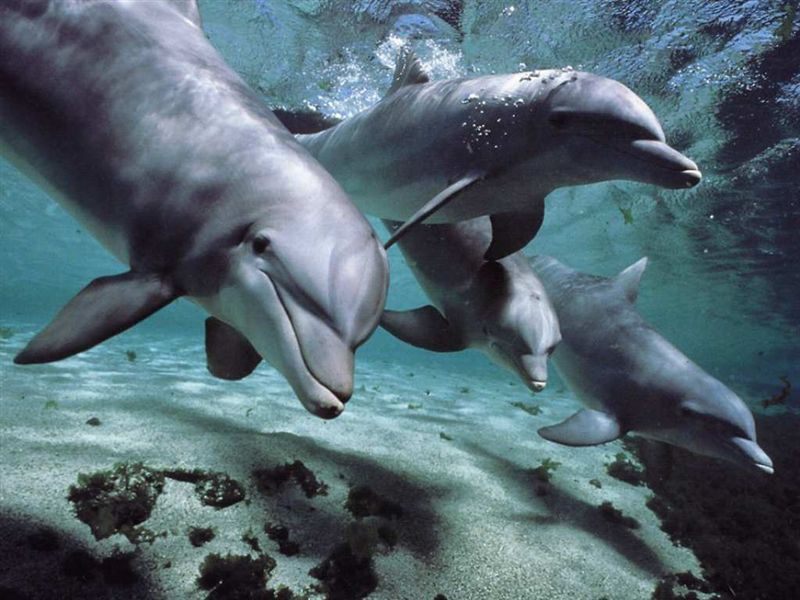This underwater photograph captures four playful dolphins swimming in shallow water from the top left towards the bottom right. The closest dolphin can be seen in the top left corner, facing towards the bottom right, looking directly at the camera. One dolphin's dorsal fin breaks the water's surface, glistening with sunlight dapples, as the dolphins move diagonally towards the bottom right corner of the frame. The seabed, only a foot or two below, is white and patterned with light and shadows, covered in patches of rocks and dark green vegetation. The colors in the image are muted and calm, with the dolphins’ skin showing a blend of gray, bluish, and purplish hues under the clear aquamarine water. Bubbles rise from the highest dolphin, adding to the sense of motion and life. The image is serene and photorealistic, capturing the joyous swim of the dolphins in a tranquil setting.